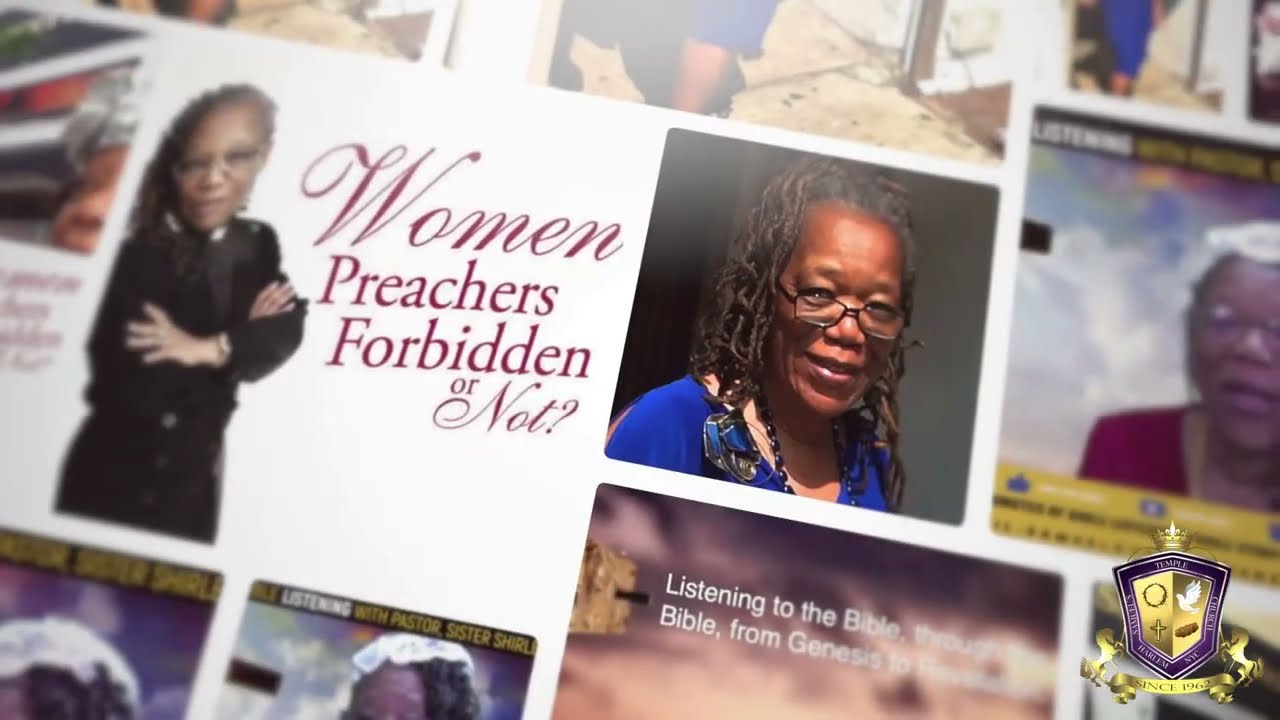This image is a collage-style arrangement of several photos and text, presented at a slight angle with a focused center and blurred edges. Each photo in the collage is outlined with a thin white border. Dominating the central area is a striking photograph of an African-American woman resembling Oprah, dressed in a black clerical suit with her arms folded across her chest. She wears black glasses, and her wavy hair cascades down her back. To the right of her image, text appears, reading "Women, Preachers, Forbidden or Not?" in a combination of cursive and print fonts, drawing a question about women in ministry. Adjacent and slightly lower, another image features an African-American woman with glasses and spiral locks drawn back from her face, perhaps an older version of the same woman. She dons a blue blouse and a black beaded necklace, with text below mentioning "Listening to the Bible, Bible from Genesis." The entire composition gives the impression of a magazine or yearbook page, partially washed out by a light source affecting its left side. In the lower right-hand corner, a prominent purple-bordered coat of arms with a golden center is adorned with a golden crown above it and a ribbon below. The coat of arms is detailed, featuring four symbols at its core and flanked by unicorns on either side of the ribbon.